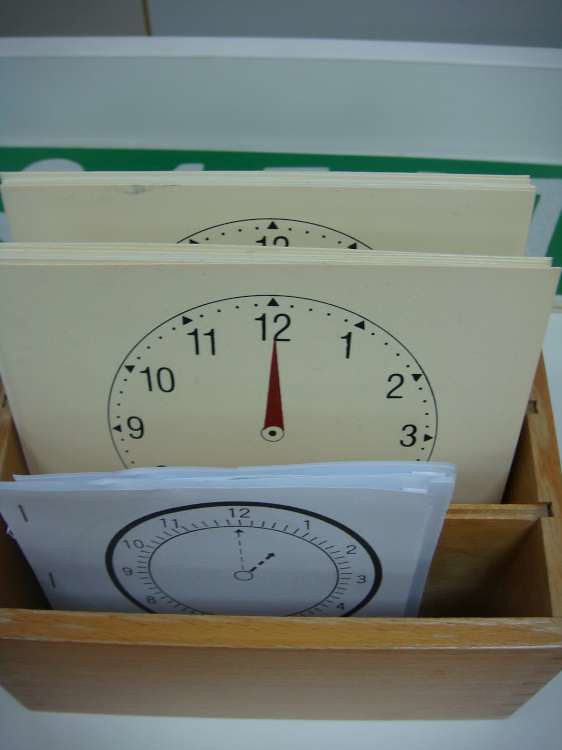This image captures a meticulously organized wooden tray seen from a top-down perspective. The tray, crafted from maple wood, contains various pictorial representations of clocks, resembling an artist’s collection of painted papers ready for review.

In the forefront, a distinctively round clock illustration is visible, marked by a bold, dark black line, with the depicted time set precisely at one o'clock. Adjacent to this, a smaller piece of paper portrays another clock illustration. This time, the paper has a subtle vanilla or beige tone. The design is minimalistic, featuring a single red, triangular clock hand pointing directly at 12, while the numerals are standard, with small arrows above each indicating their positions.

Nestled behind these prominent papers, there appears to be another stack, hinting at a duplicate set of illustrations. Additionally, a partially obscured green and white sign is visible behind the papers, with only the tops of the letters discernible, rendering the text illegible.

The layout within the tray is organized into three distinct sections, each housing the various clock-themed papers, contributing to a sense of structured artistic arrangement.